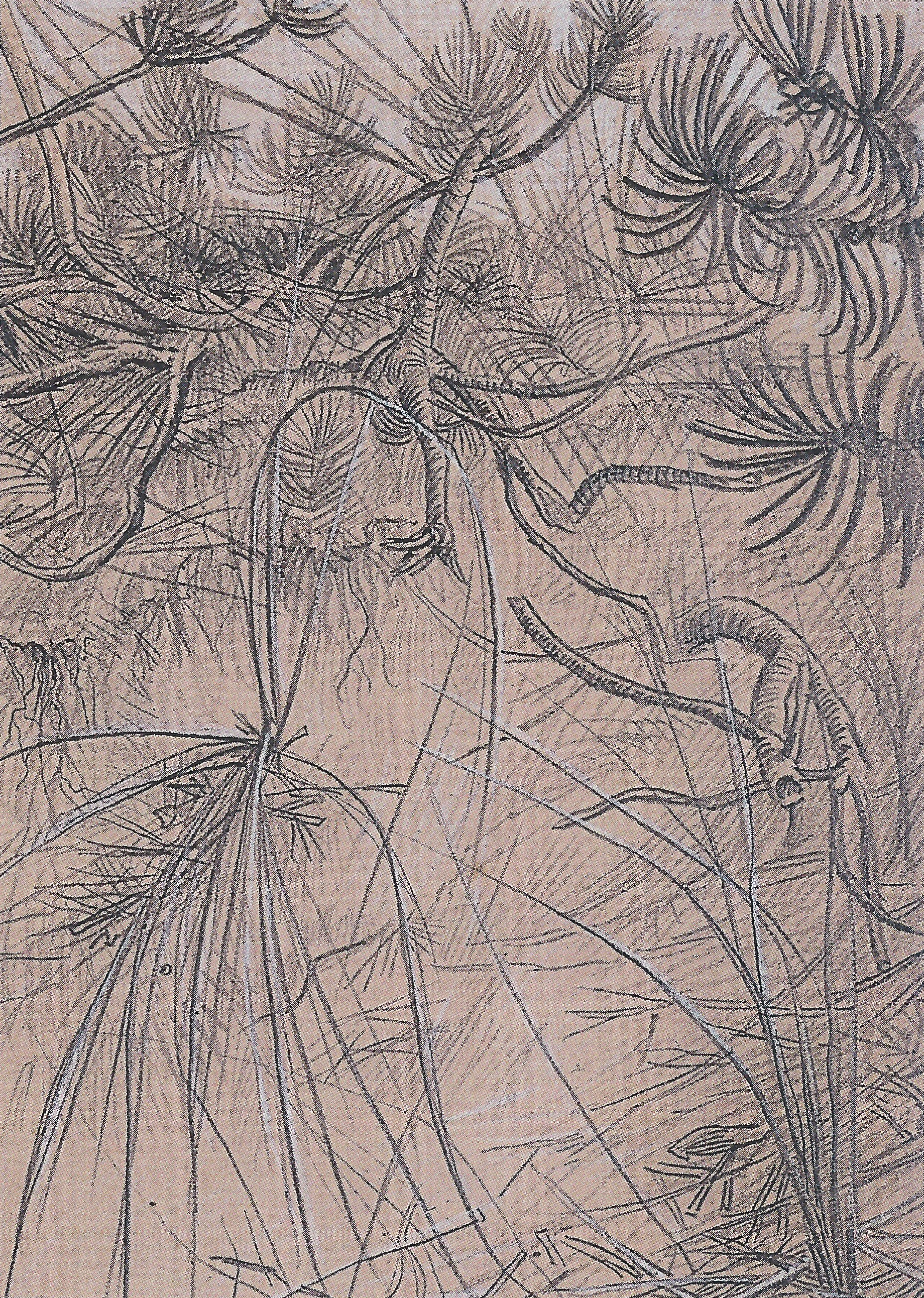The image is a tall, rectangular pencil drawing on light tan construction paper, seemingly depicting an aerial view of a dense, leafless forest or a complex network of twisting and tangling branches. The background gradient transitions from a lighter gray at the top to a more tannish hue towards the bottom. The drawing, predominantly consisting of various shades of dark gray, features an intricate mesh of branch-like structures, with some elements resembling pseudo-fern-like shapes or coral formations. Throughout the composition, branches and sticks crisscross and intertwine, creating a textured, sketchy appearance. The detailed lines vary in thickness, achieving a sense of depth and shading that enhances the intertwining forms as they spread randomly across the scene.